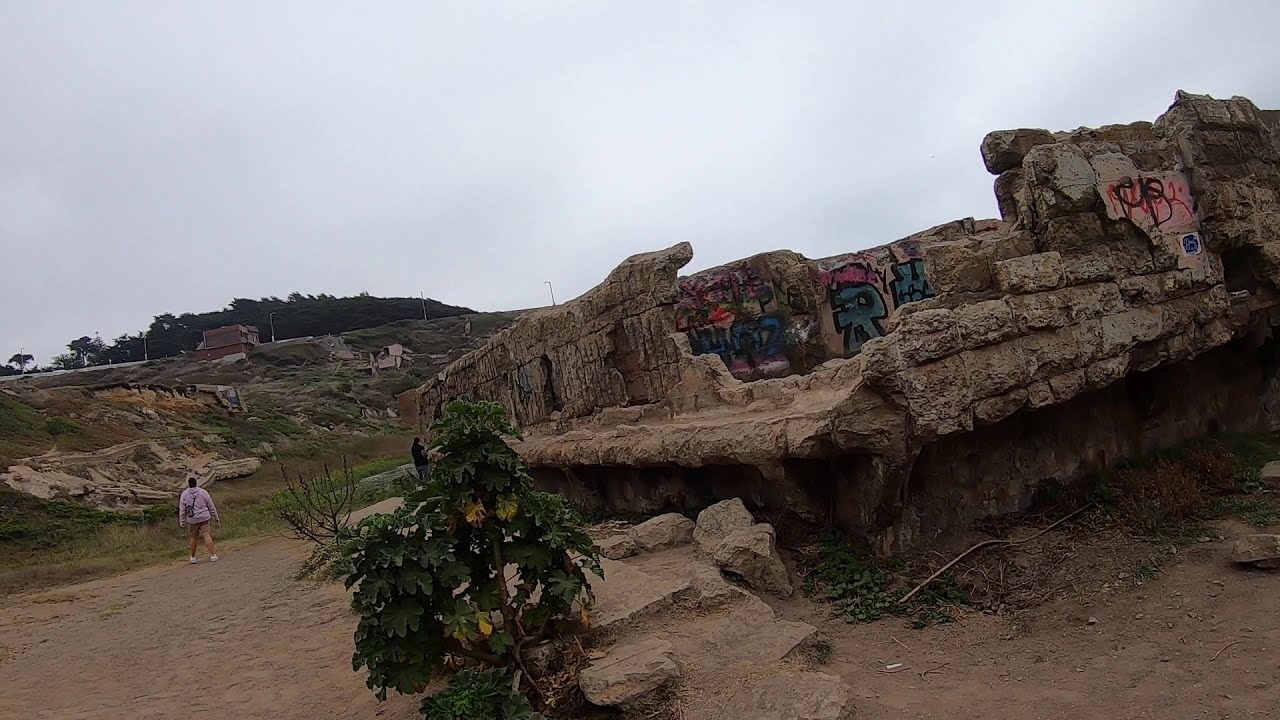The photograph is a horizontally aligned rectangular image taken outdoors, featuring a striking, partially destroyed rock structure. The overcast sky, blending gray and white clouds, forms the backdrop in the upper part of the image. The middle section, especially on the right, is dominated by the rock structure, which appears to have once been a building. Large brownstones are stacked upon each other, creating a wall that has now partially crumbled. This aged structure is adorned with graffiti, including prominent blue letters outlined in black, along with splashes of pink and purple paint. 

The ground beneath is mostly dirt, scattered with small rocks and patches of weeds and grass. On the middle left, a small tree or bush with green leaves can be seen. Toward the lower left side of the image, a woman in a pink hoodie stands on the dirt ground. She appears slightly heavyset, with a bag slung around her left shoulder, and is looking up a slight incline leading to a distant hilltop, where a building and streetlights are visible, indicating the presence of a road.